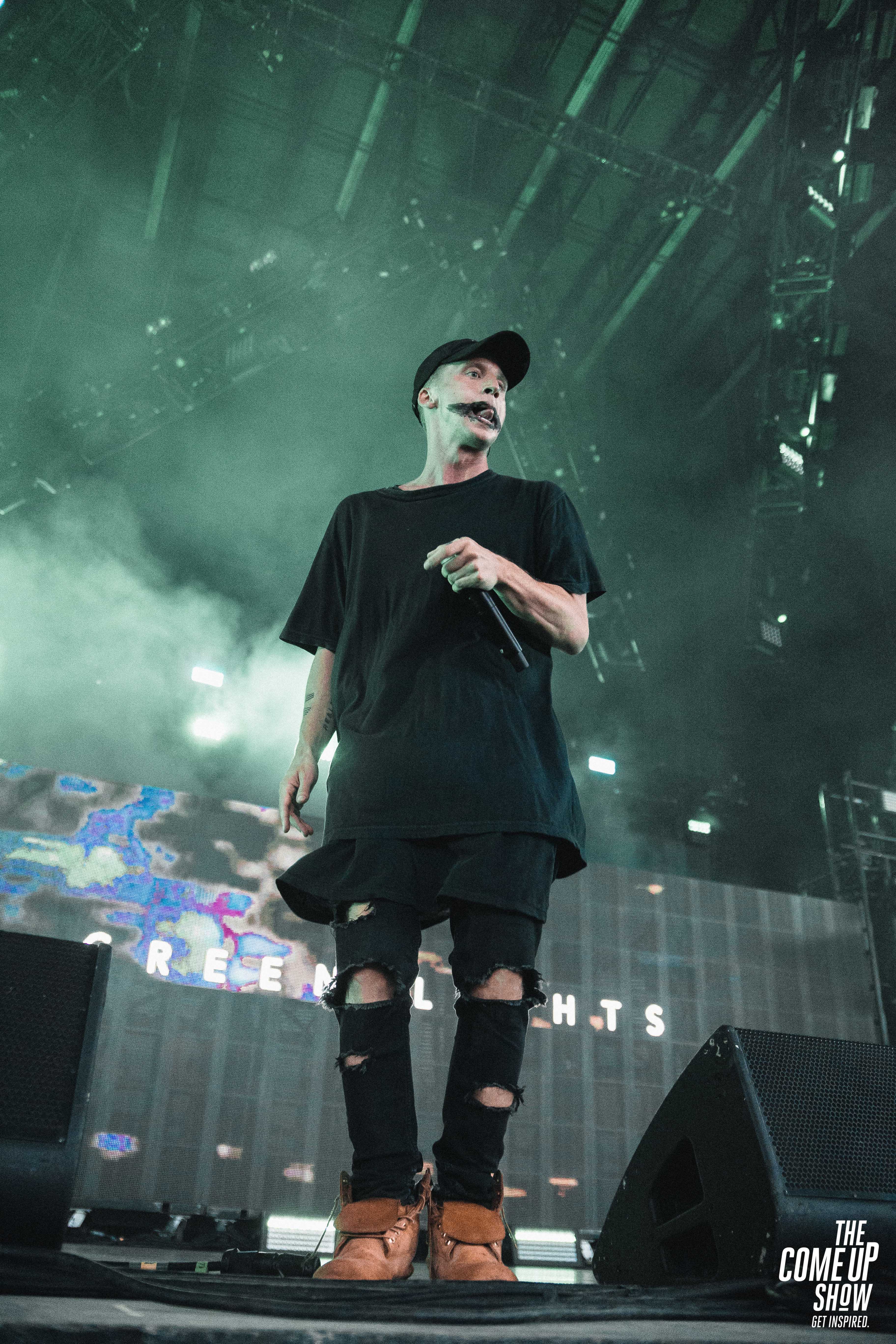This captivating image depicts a man performing on a stage, taken from a low angle that emphasizes the grandeur of the setting. He appears to be in his twenties, with a Caucasian complexion, a shaved head, and a clean-shaven face highlighted by striking black makeup around his mouth. Adding to his enigmatic presence, he's sticking his tongue out slightly. His attire is predominantly black, including a black baseball cap, a layered oversized black t-shirt, and black jeans with numerous rips, showcasing a rebellious style. Finishing off his outfit, he's wearing untied brown boots that hang loosely around his feet.

The stage is set in a vibrant and somewhat industrial environment, with steel girders and beams visible over his head, adding a sense of structure and depth. There's also mysterious, greenish-white smoke swirling in the air, lending an atmospheric touch. Hanging from the ceiling, a clear, undefined object adds a curious element to the scene. The background is dark, with some sound equipment and speakers flanking him, and partially visible text on either side spelling out "R-E-E" on one part and "H-T-S" on the other. At the bottom right corner of the image, white print reads "The Come Up Show - Get Inspired," indicating the possible event or program he is partaking in. The visual elements combine to convey an intense and highly stylized performance setting, drawing viewers into the dynamic world of the performer.